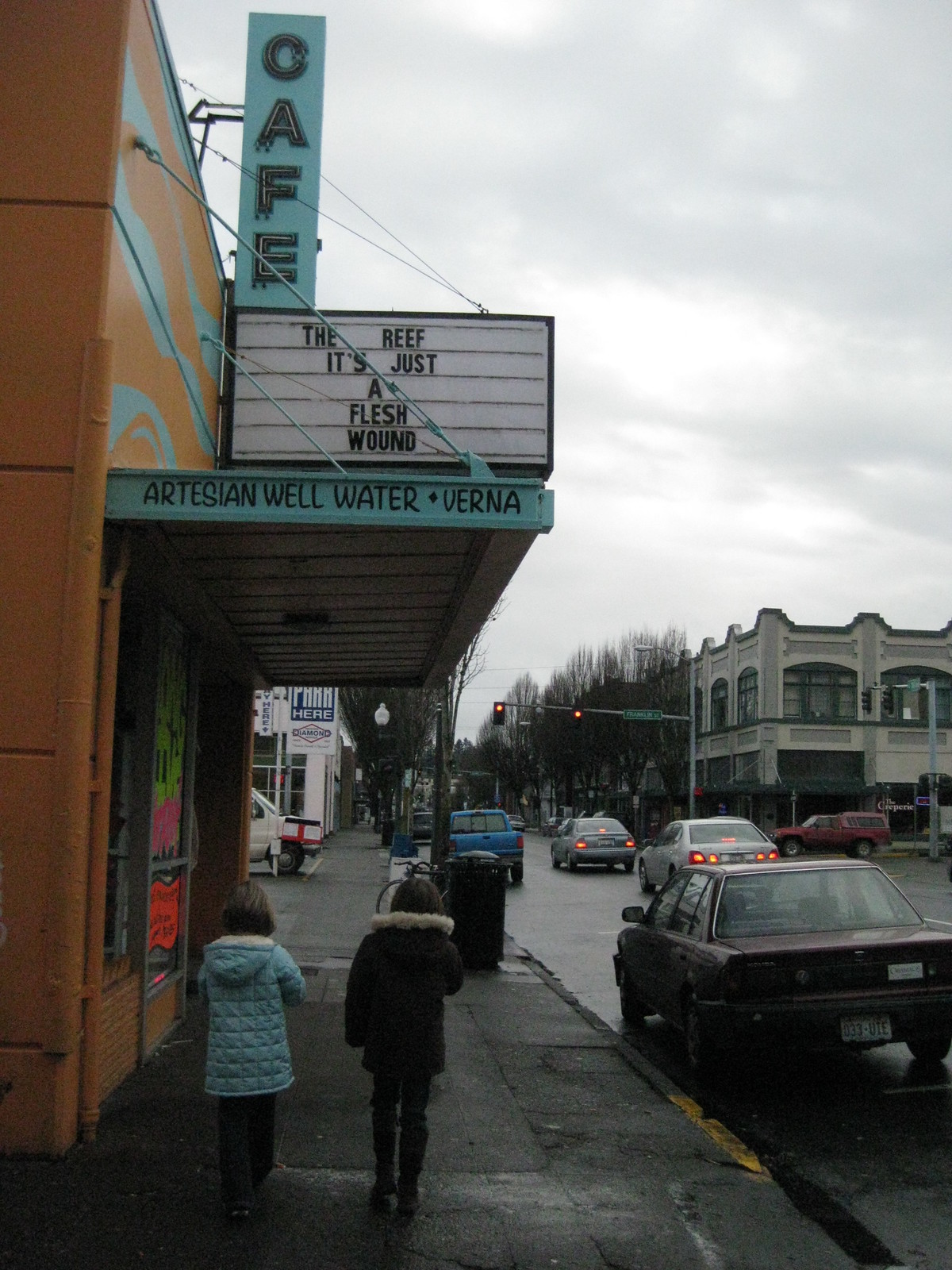In this detailed image, a bustling street scene is captured with an emphasis on an orange cafe with teal trim, located on the left side of the photo. The cafe's sign displays "Cafe" atop a blue sign that reads "The Reef. It's Just a Flesh Wound," followed by, "Artist in Well Water, Verna." The street bustles with several vehicles, including a blue Ford Ranger and a dark burgundy car parked beside the sidewalk, a white van in the distance, and at least two silver cars along with a dark red truck with a camper top stopped at a red traffic light. 

The backdrop features a large gray building with dark green trim and an overcast gray sky filled with dense clouds. Two children are walking away from the camera, appearing to head towards the cafe. The child on the left, with short brown hair, is dressed in a light blue coat with a hood, dark pants, and dark shoes. The child on the right, sporting a black coat with a fur-trimmed hood, black pants, and black shoes, also has dark brown hair. Surrounding the scene, bare trees indicate a cold day, further emphasized by the winter attire of the children. The overall setting evokes an older urban area, reminiscent of upstate New York.